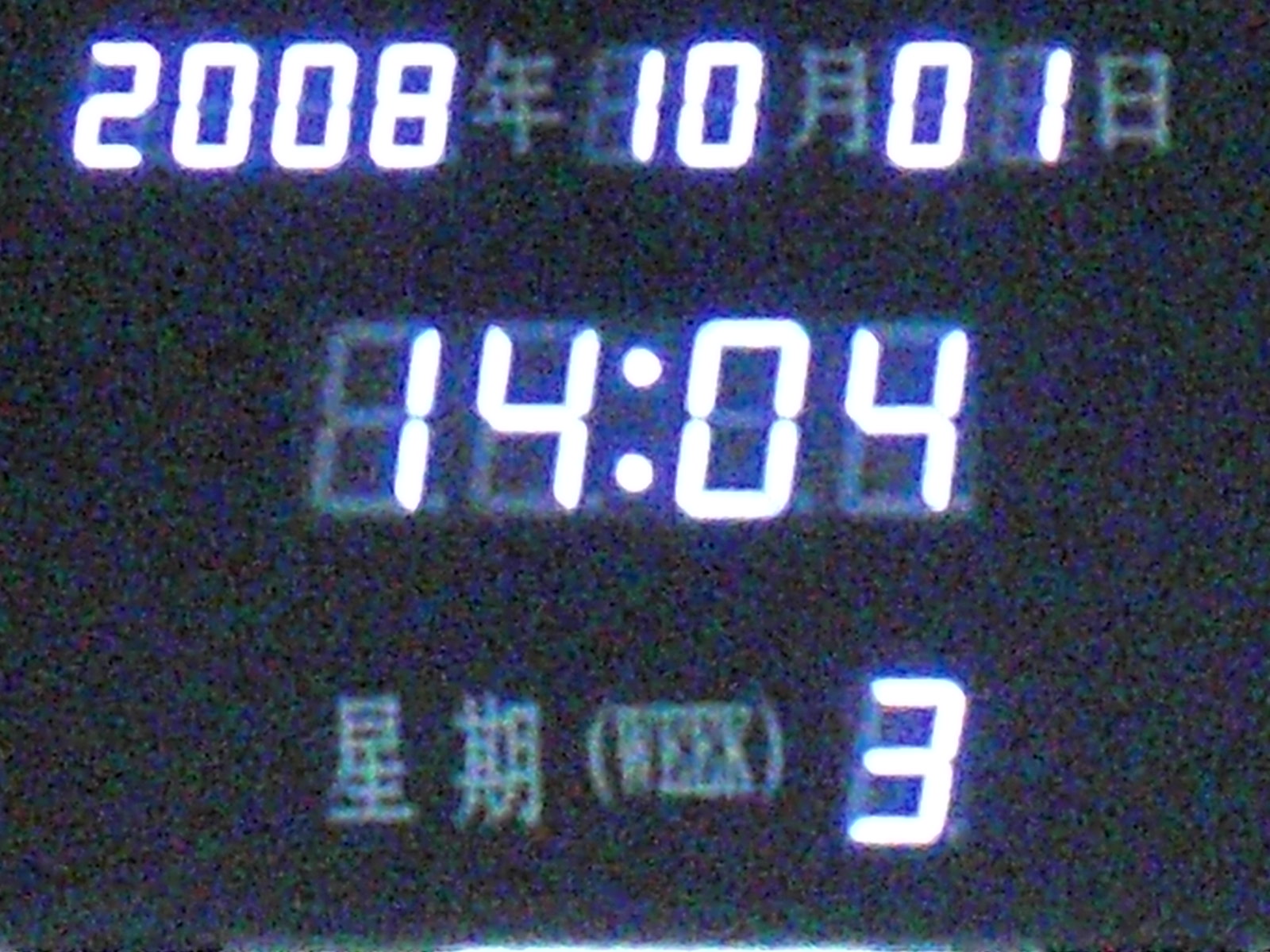The image is horizontally oriented with a black background, characterized by hazy and blurry blue, purple, and green pixelations. Prominently displayed in white LED-style digits with a faint blue glow, the text is organized into three rows. The top row reads "2008年10月01日," denoting the year, month, and day, separated by Chinese characters for "year," "month," and "day." The middle row shows "14:04," indicating the time of 2:04 PM. The bottom row features two Chinese characters followed by the English word "week" in parentheses and the number "3," suggesting it is the third day of the week.